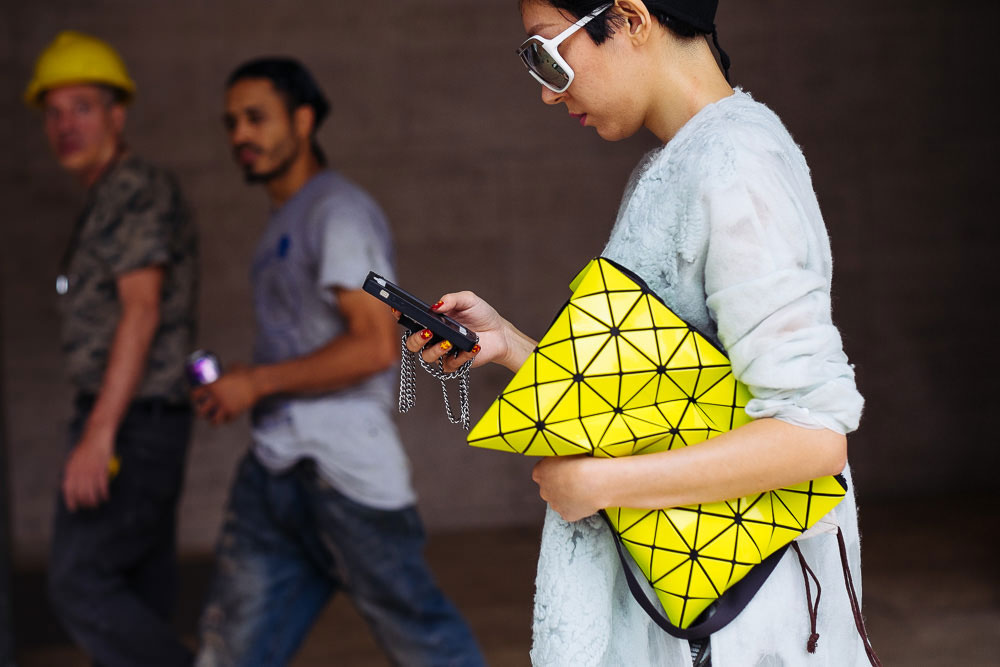In this professional outdoor photo, a Caucasian woman with short brown hair, styled with a rat tail, stands in the foreground under a building awning, engrossed in her black smartphone. She has striking red fingernails and wears large white sunglasses. Her attire consists of a light blue dress or a long-sleeved white shirt rolled up to her elbows, and she holds a bright yellow rectangular purse adorned with a geometric pattern of black lines and squares under her left arm. The blurred concrete background features a white stone wall, and two men walk beside her, moving to the left. One man, older and Caucasian, wears a yellow construction helmet, a camo short-sleeved shirt, and blue jeans. The other man, younger and African American, dressed in a gray t-shirt and blue jeans, holds a can of soda and sports a goatee.